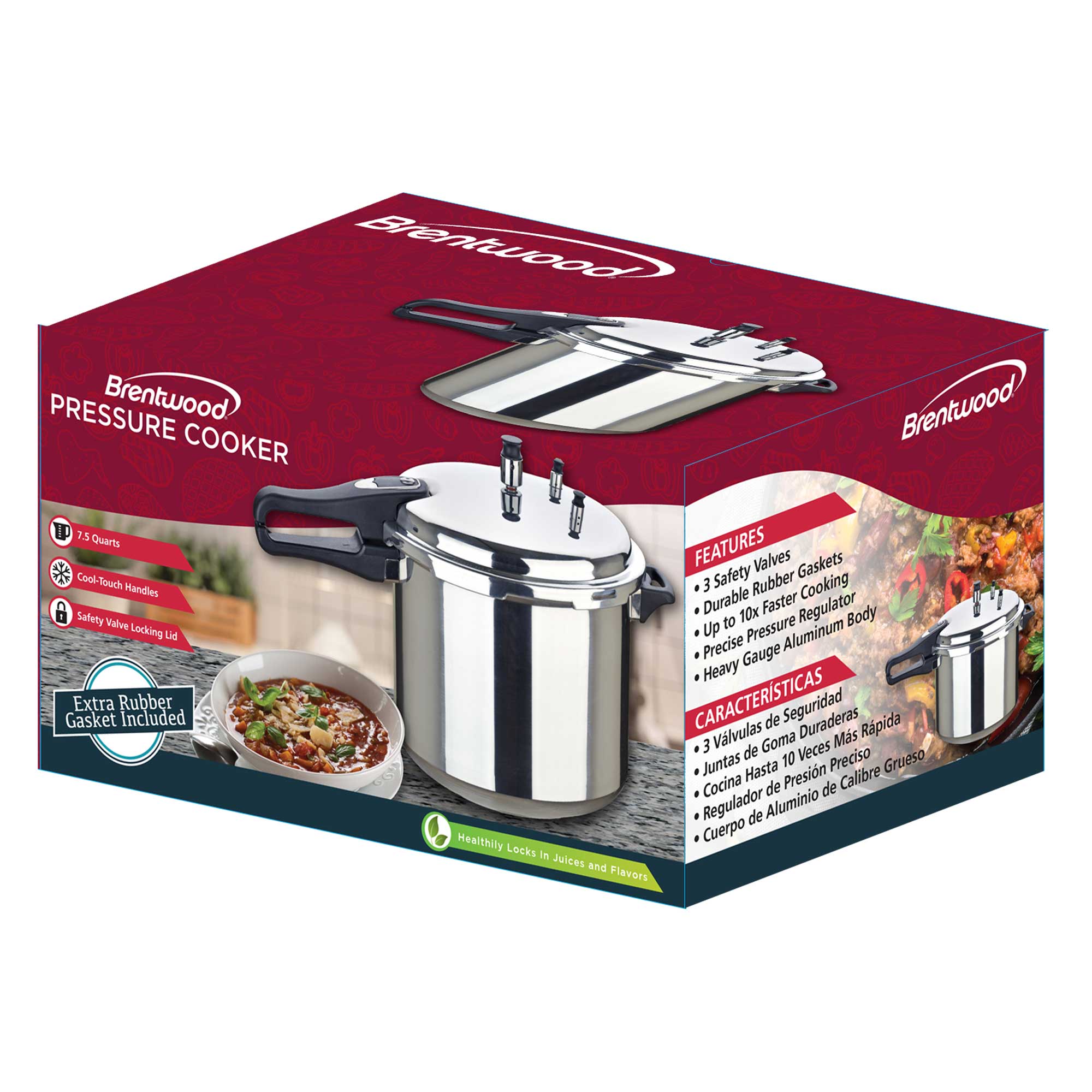This color photograph is taken slightly above the product packaging of a Brentwood pressure cooker, showcasing the top and two sides of the box. The main color of the top of the box is a plum or maroon red with "Brentwood" written in bold white letters. The pressure cooker, prominently featured in silver metal with a large black handle and steam escape prongs, is visible on all three sides of the packaging. A white bowl of chili, presumably made with the pressure cooker, is illustrated on the sides of the box, set against a backdrop of grey countertops.

On one side of the box, there are five bullet points in black text on a white background, detailing the pressure cooker's features: three safety valves, durable rubber gaskets, up to ten times faster cooking, a precise pressure regulator, and a heavy gauge aluminum body. These features are also repeated in Spanish. Additionally, the packaging highlights an extra rubber gasket included and an environmentally friendly label on the bottom right.